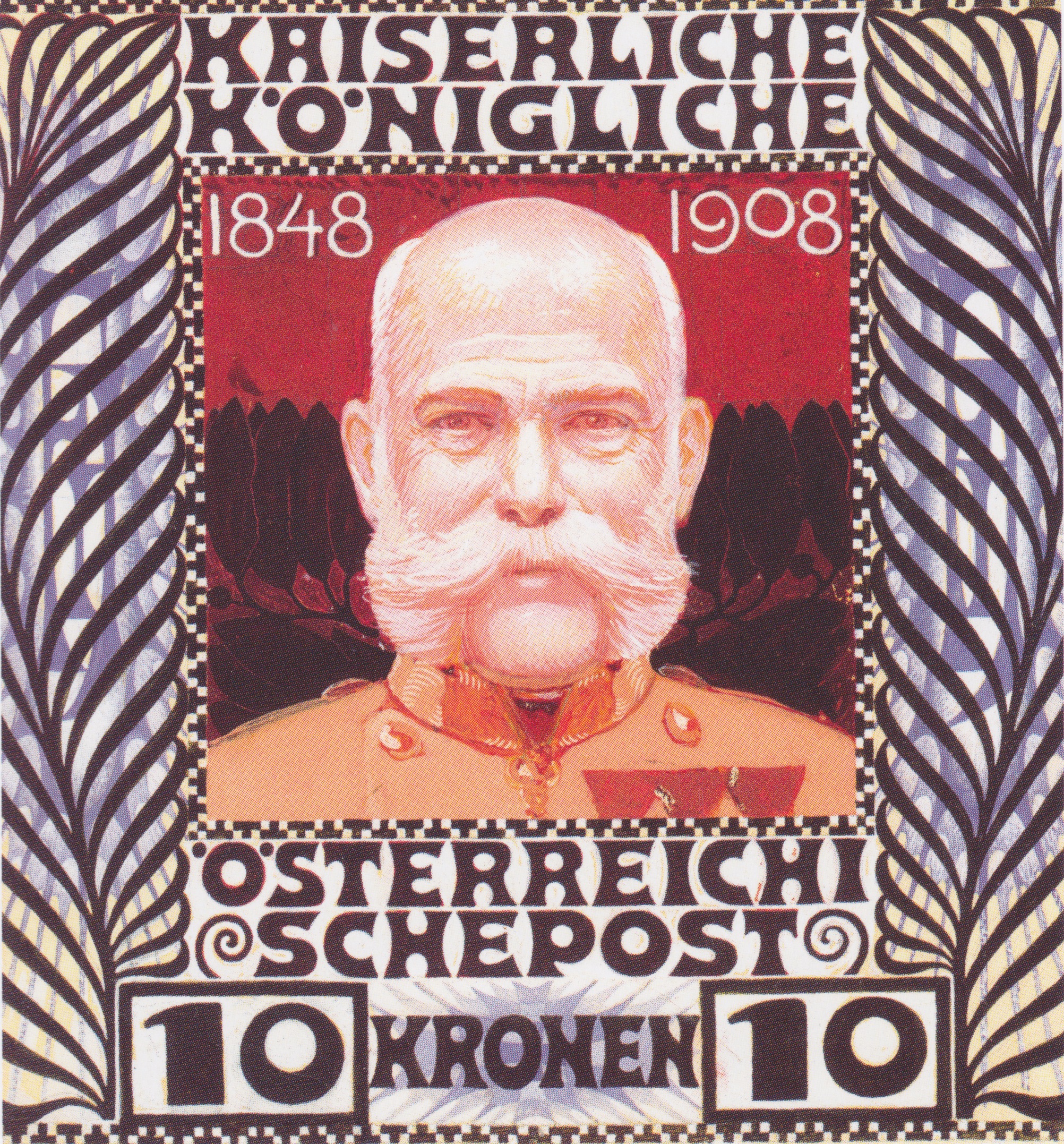This is a detailed depiction of a tall rectangular stamp bearing elaborate designs. At the top, within a white rectangle and in a fancy font, it reads "Kaiserlich Königlich." Centered is a square portrait of an old man who is bald with white hair on the sides, a prominent white mustache, and a beard that outlines his face but leaves his chin bare. He gazes straight ahead, adorned in what appears to be an orange military uniform. Just above his head, the stamp features the dates "1848" on the top left and "1908" on the top right, set against a red sky with black tree-like imagery in the background. Below the portrait, it reads "Österreichische Post 10 Kronen 10," framed by ornate black, blue, and white floral and linear patterns. The intricate detailing and foreign text suggest it is an old, possibly European, stamp, rich with historical connotations.